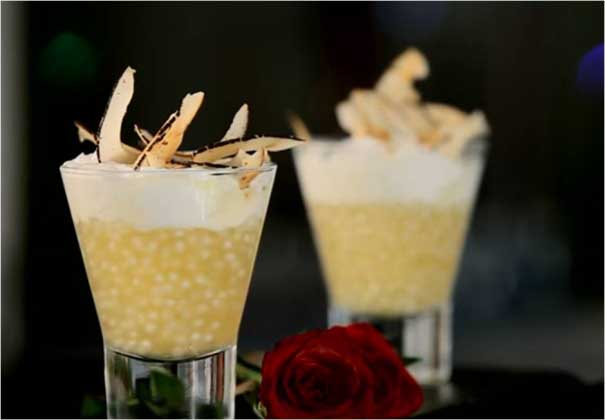The image showcases two unique mixed drinks presented in glasses that possess a wide, conical top tapering into a thick, clear cylindrical base. Each glass contains a layered beverage, with a base of pale yellow liquid embedded with tiny white balls, likely tapioca pearls, topped with a generous layer of white cream. Garnishing the cream topping, there are shavings that resemble either lightly burned edges of white chips or perhaps toasted coconut or almond flakes—adding an appealing texture and visual contrast. Resting in front of these aesthetically crafted drinks is a single red rose, lying gracefully on a sleek black table that reflects no light, emphasizing its color and form. The background of the image appears dark and softly mottled, slightly out of focus, providing a striking yet unobtrusive backdrop to the elegant arrangement in the foreground.